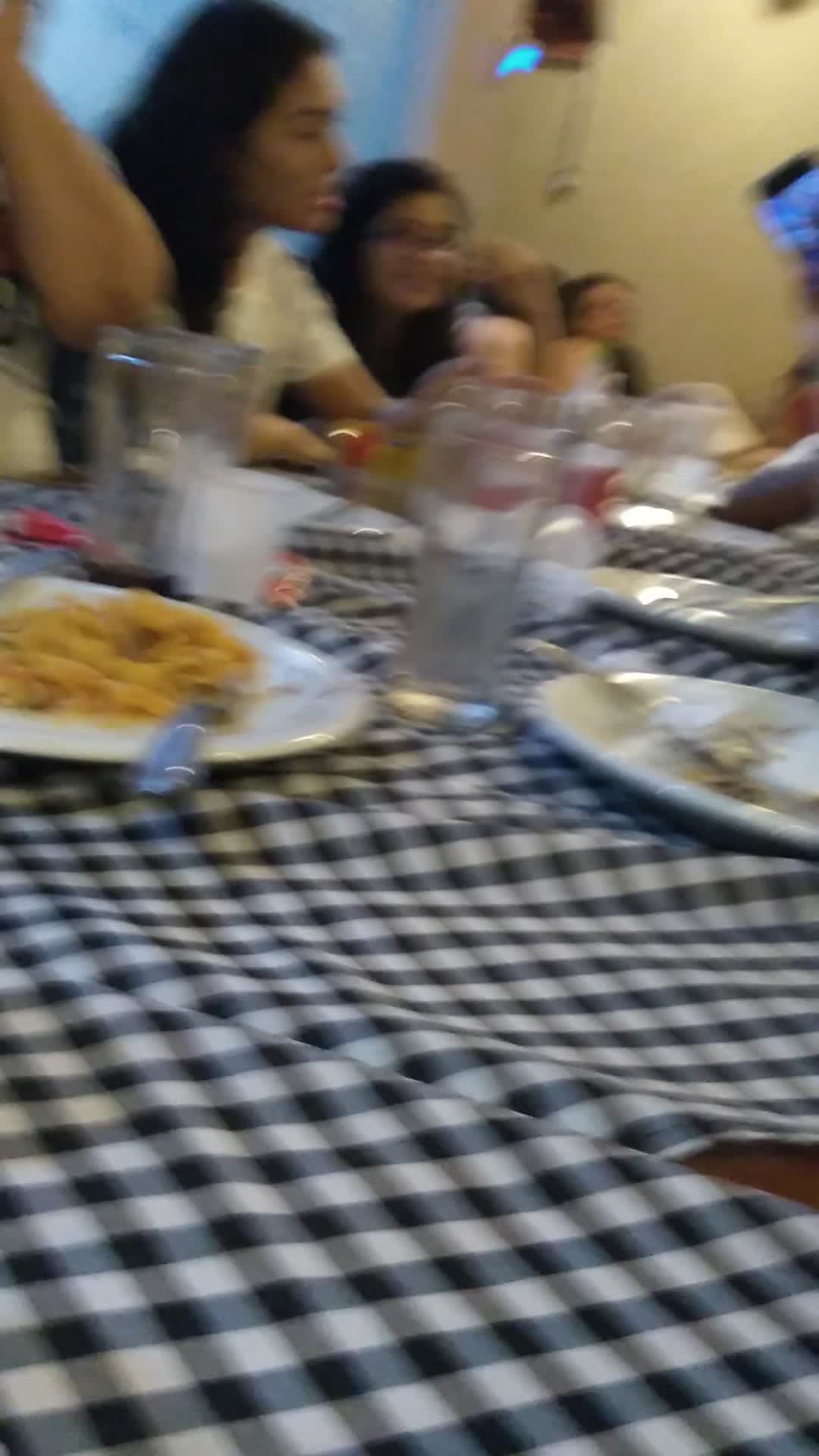This blurry indoor photograph captures an evening of dining and conversation, possibly in a home or a restaurant setting. Centered around a long rectangular table draped in a black, white, and gray checkered tablecloth that appears gathered and uneven, the image shows a row of five people—mostly women—on one side of the table. Among them, two girls with long black hair are prominently visible, with one facing the camera. The table is adorned with several plates containing remnants of food, clear water glasses, napkins, and part of a smartphone being held by someone whose face is out of the frame. The background features a tan wall with a window in the upper left corner. Despite the photo's poor focus, it suggests a warm atmosphere where people are enjoying each other's company and engaging in lively conversation.